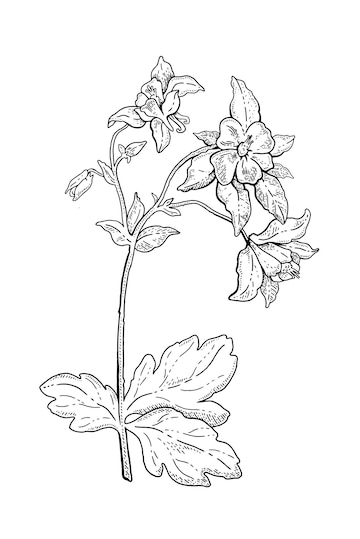This black and white illustration resembles an image from an old coloring book or a botanical guide. It features a single flowering plant, with multiple thin stems extending upward and outward. The base of the plant is adorned with three large leaves that resemble elm tree leaves. Moving upward, there are a few smaller teardrop-shaped leaves dispersed along the stems. The central stem rises vertically bearing a fully bloomed flower at its tip. To the right, another branch extends laterally, presenting two fully bloomed flowers and one bud-like structure that is partially obscured by leaves. The flowers each display four petals with a distinct center. The entire illustration is set against a white background, emphasizing the simplicity and elegance of the plant's form.